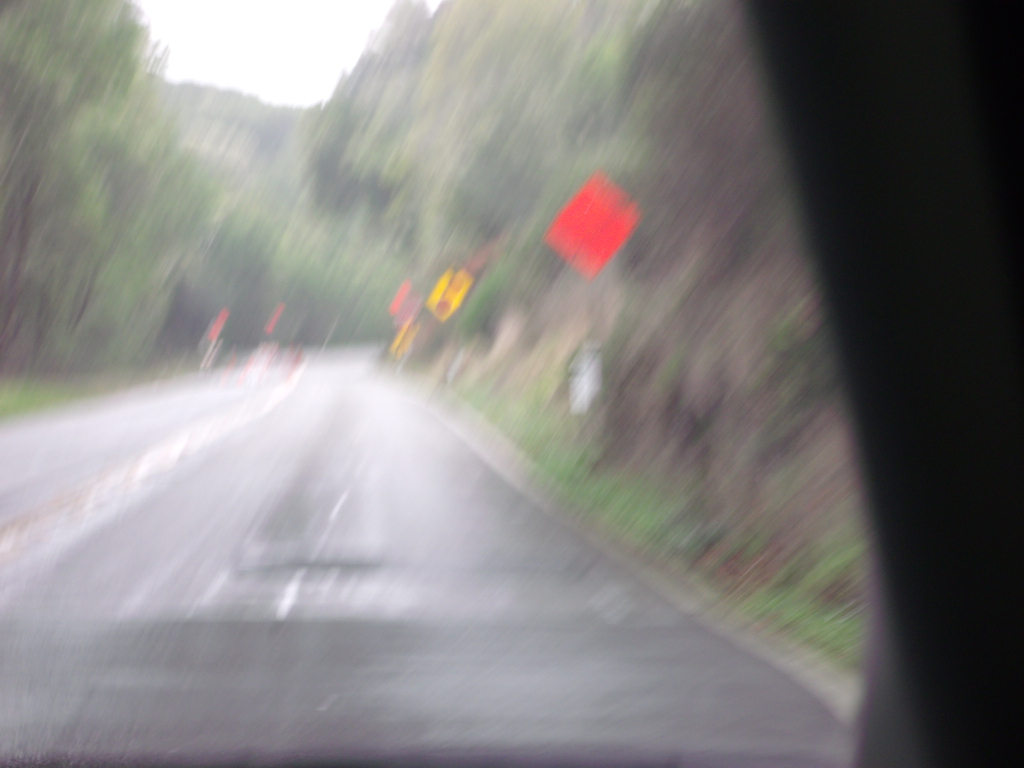This blurry photograph captures a curving country road framed by lush greenery, as if taken from within a moving vehicle. The gray asphalt road extends forward before disappearing around a bend, creating a sense of journey and mystery. To the right, a steep, verdant hill is adorned with grass, trees, and shrubs, contributing to the natural landscape. On the left side, a dense line of green trees forms a picturesque boundary. Various road signs punctuate the scene: a red diamond-shaped sign on the right, though its text isn't discernible, followed by a yellow sign further down. Even farther, near the bend, red signs are visible on both sides of the road, adding a splash of color to the green-dominated scenery.